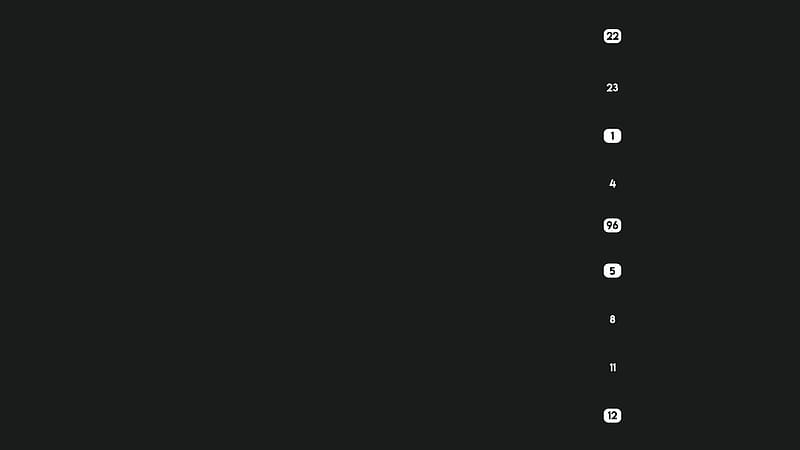The image is predominantly a solid black rectangle. Roughly 80% of the way across from the left, there is a column of numbers extending vertically down the right-hand side. These numbers alternate between white text directly on the black background and black text inside white squares. Starting from the top, the sequence is as follows: a white square with the number 22 in black, the number 23 in white, a white square with the number 1 in black, the number 4 in white, a white square with the number 96 in black, a white square with the number 5 in black, the number 8 in white, the number 11 in white, and finally, a white square with the number 12 in black. There are no other elements in the image.